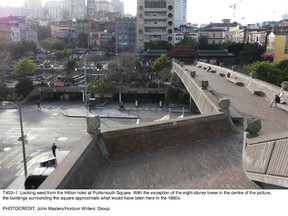The image depicts an outdoor urban scene in a landscape layout, featuring a concrete overpass that spans a street or roadway. Below the overpass, trees and a few pedestrians are visible. Above the overpass, the background comprises a mix of tall buildings, including what appear to be apartment and commercial structures, some possibly situated on hills, creating a varied skyline. The scene is set during the daytime, and flags can be seen fluttering atop some buildings, suggesting it might be in a foreign country. Alongside the detailed urban landscape, the image includes a small, blurry section of black text at the bottom, which is difficult to read. The overall perspective offers a sense of depth with a populated area in the distance and a large courtyard or park area below the overpass.